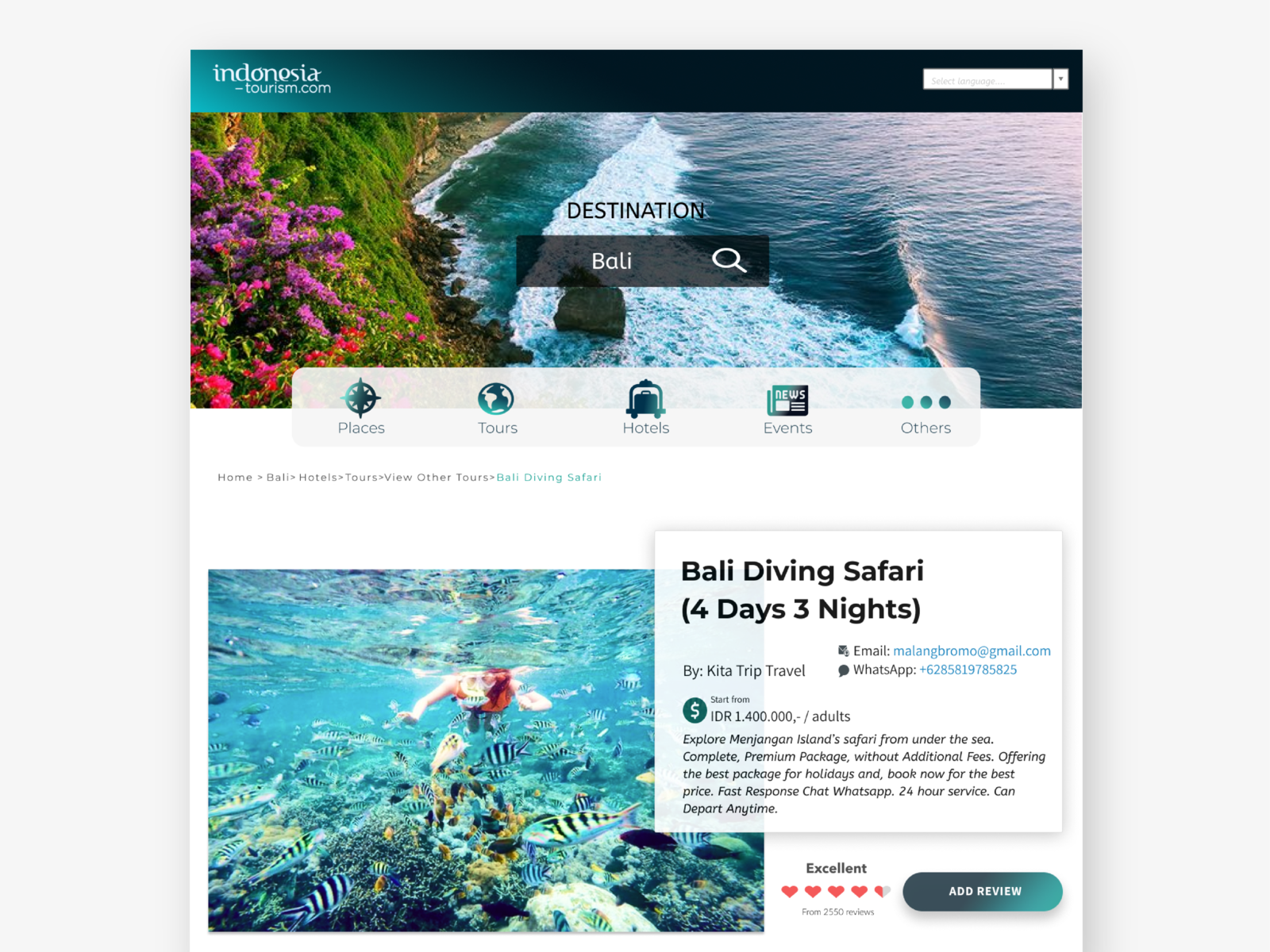Certainly! Here's a detailed and cleaned-up caption:

---

This image captures a screenshot of what appears to be a template for a tourism website, indonesiatourism.com, though it could also be the actual site. The screenshot has been enhanced with a drop shadow, giving it a polished look. 

At the top of the page, there's a striking hero image showcasing a stunning cliff adorned with vibrant purple and red flowers. Below the cliff lies a rocky coastline transitioning into a sandy beach, with waves gently rolling in from the right. The serene ocean gleams beautifully under the sunlight coming from the upper right corner, creating a picturesque scene. 

In the upper right section of the header bar, there's a search field. Superimposed on the hero image are the words "Destination" and a black search field labeled "Bali" featuring a magnifying glass icon. 

Beneath this, the website offers five icons representing different sections: Places, Tours, Hotels, Events, and Other. These icons are designed as a navigation compass, a globe, a suitcase on a bellhop cart, a newspaper, and three dots respectively.

Further down the page, there's an image of a diver exploring a shallow reef teeming with hundreds of colorful fish. The diver, equipped with a mask, is captioned by "Bali Diving Safari," detailing an adventure package lasting four days and three nights. The cost is displayed as IDR 1,400,000 (Indonesian Rupiah), though the exact amount may be clarified. 

Additional features include the option to email or use WhatsApp for inquiries, a rating of four and a half hearts, and an "Add a Review" button. Below the price, there is some explanatory text for further clarification.

---